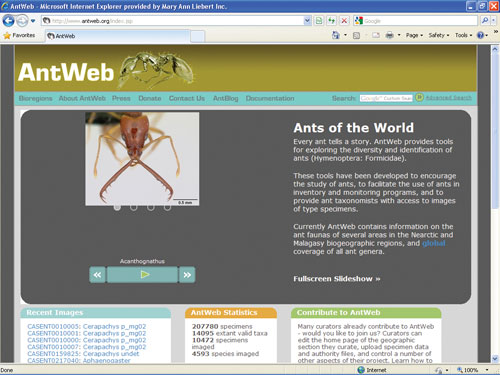The screenshot features a webpage from AntWeb, an educational platform dedicated to ant species identification, presented through what appears to be an old-school Microsoft Internet Explorer browser interface provided by Mary and Webert Inc. At the top of the browser, black text indicates "AntWeb," and the standard browser controls are visible on the right side, including the minimize button, another unidentified button, and the red 'X' close button. 

The browser toolbar showcases typical Internet Explorer buttons such as a blue arrow pointing right, a green arrow pointing left, a refresh icon, and a Google search bar integrated under every page. Additional buttons for managing favorites and open tabs are also present.

The AntWeb website header features the name "Web Ant" in white Varnish font, accompanied by an image of a brown ant against a gray background. The main navigation menu includes links to About, Press, Donate, Contact Us, Ant Blog, and Documentation, along with another Google search box. Another image of a brown ant is displayed under the navigation bar.

On the right side of the page, a tagline reads, "Answer the world, every ant tells a story," and the text outlines that AntWeb provides tools for the exploration and identification of ants. These tools are designed to encourage the study of ants and their incorporation into inventory and monitoring systems. The text further details that AntWeb offers access to type specimens and relevant images, currently containing information about ant farms in several areas of the Netherlands, with a note on its global coverage.

Towards the bottom of the page, there are sections for recent images, though they are not displaying, along with information on the number of species cataloged and contributors to the platform.